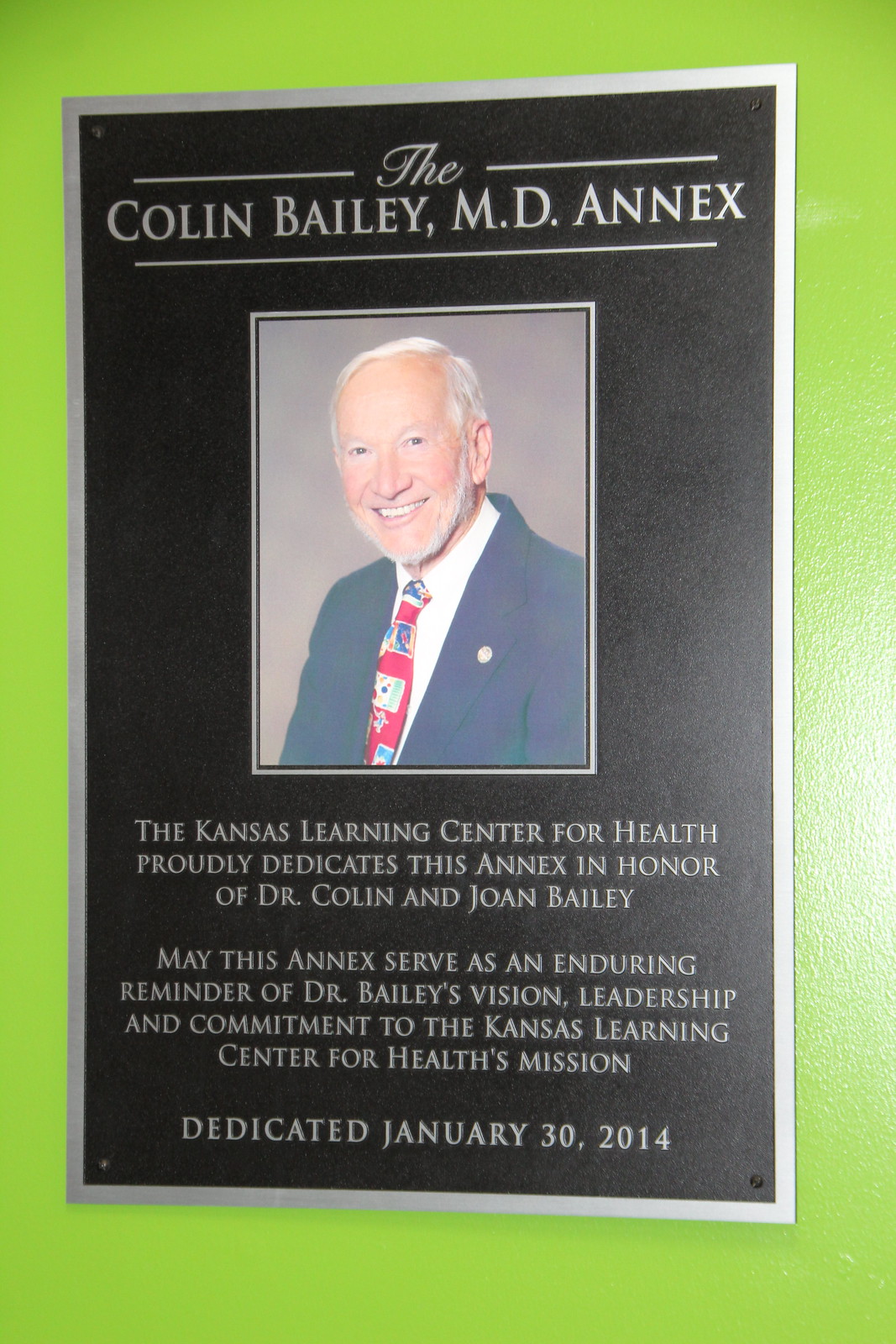The image showcases a rectangular dedication plaque with a silver frame and a black background, prominently displayed on a lime green wall. At the top of the plaque, the text reads, "Dr. Colin Bailey, MD, Annex." Below this title, there is a smiling photograph of an older man with white hair and a white beard, dressed in a dark jacket, a white shirt, and a vibrant, patterned red tie. The inscription beneath the photograph states, "The Kansas Learning Center for Health proudly dedicates this annex in honor of Dr. Colin and Joanne Bailey. May this annex serve as an enduring reminder of Dr. Bailey's vision, leadership, and commitment to the Kansas Learning Center for Health's mission. Dedicated January 30, 2014." A light source illuminates the plaque from the right side, enhancing its visibility on the green wall.